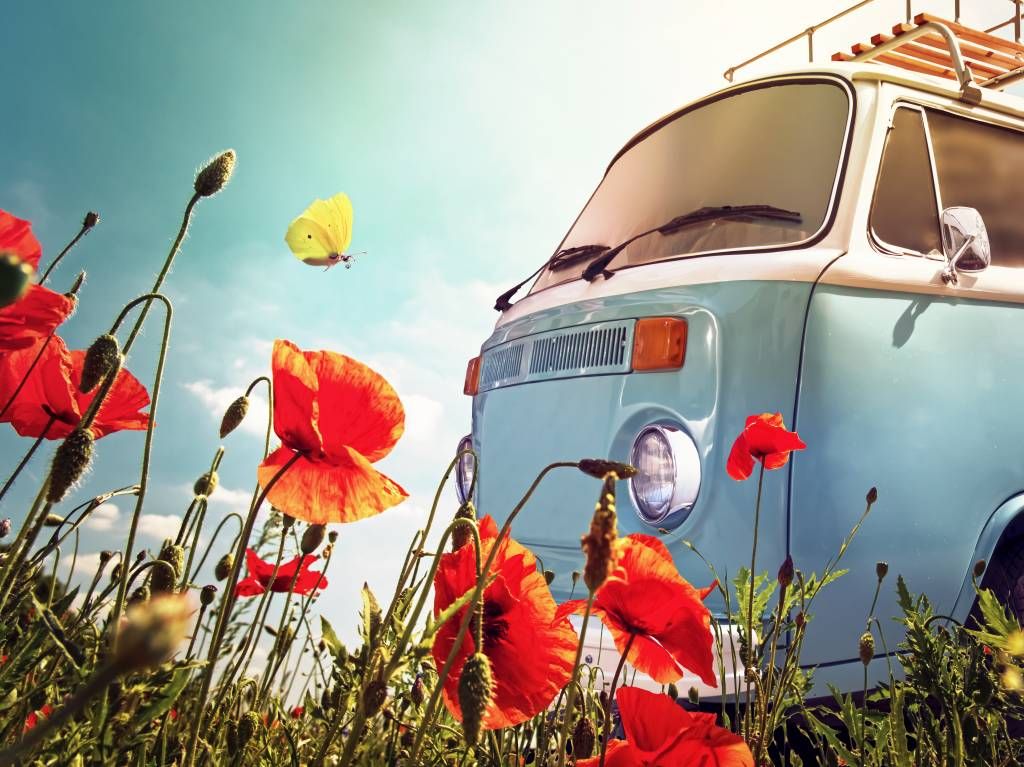This vibrant photograph captures a striking blue and white Volkswagen van, likely vintage, with a wooden luggage basket on its roof, situated in the middle of a lush, grassy field. The photo is taken from a low, ground-level perspective, looking up through a dazzling foreground of orange poppies, scattered wild red and yellow flowers, and abundant green grass. The front portion of the van dominates the right-hand side of the image, showcasing its flat nose, headlights, grill, tinted windshield, and distinctive orange marker lights. Above the flowers, a delicate yellow butterfly flutters near the van's front. The backdrop features a bright, blue sky filled with clusters of white clouds, framing the gleaming and well-maintained vehicle, with sunlight subtly highlighting its polished surface. The scene blends natural beauty with the timeless charm of the classic Volkswagen, creating a picturesque and nostalgic moment.